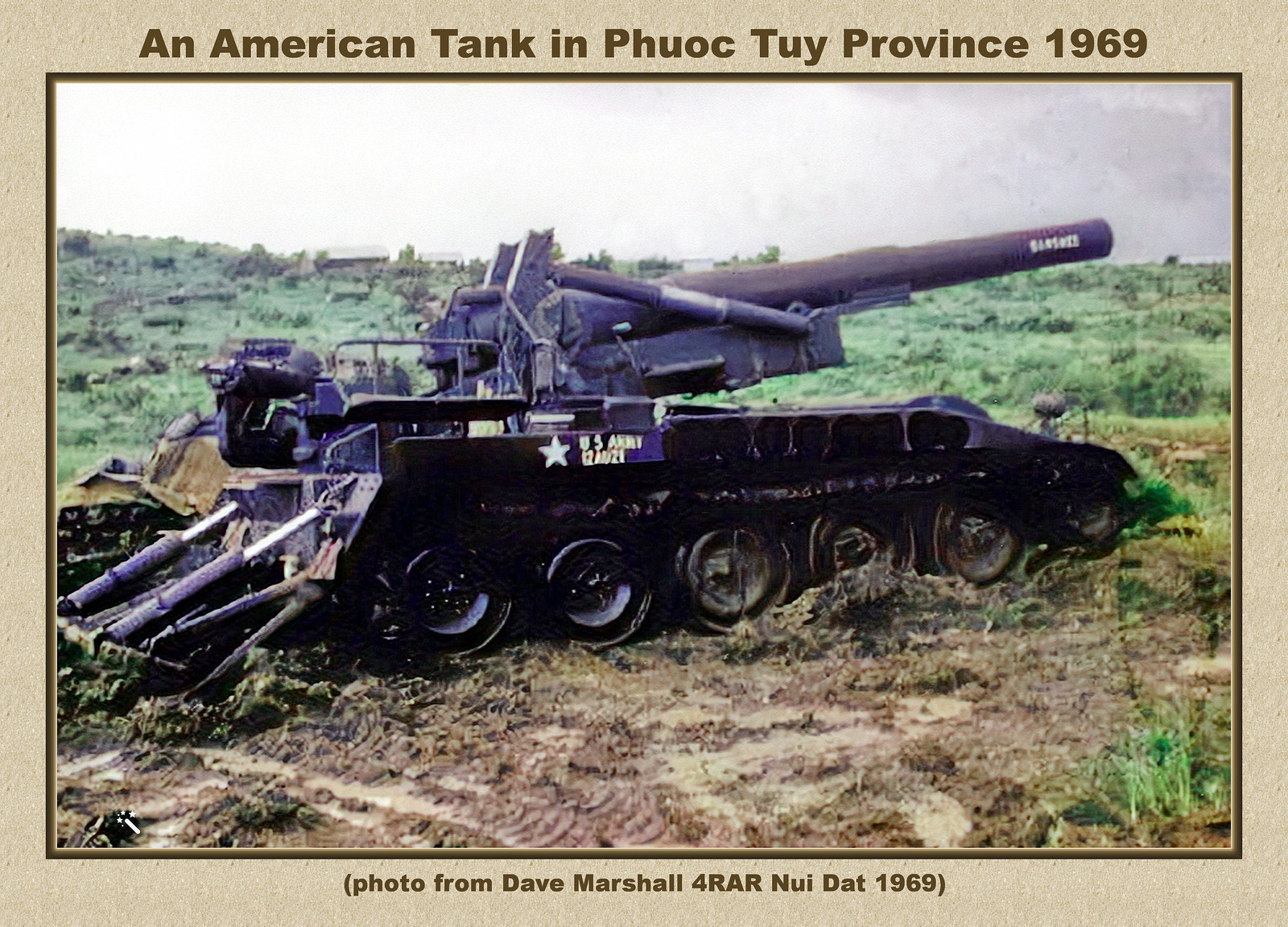The image depicts a large, black, vintage military tank situated in the center of a dirt and grassy field, characterized by visible tire tracks that suggest the tank has recently traversed the area. The tank has a star emblem on its side, marked with "U.S. Army" and additional letters and numbers. Notably, there are six tires on each side of the vehicle. The backdrop reveals a cloudy sky, distant trees, grassy expanses, and a few buildings on the horizon.

The entire picture is framed with a tan border containing text: at the top, it reads "American Tank in Phuoc Tuy Province, 1969," and at the bottom, it states "Photo from Dave Marshall, 4 RAR, Nui Dat, 1969." The setting appears to be in Vietnam, during the daytime, with no people present in or around the tank. The prominent colors in the scene include various shades of tan, brown, green, gray, and black, adding a muted, historical ambiance to the photograph.